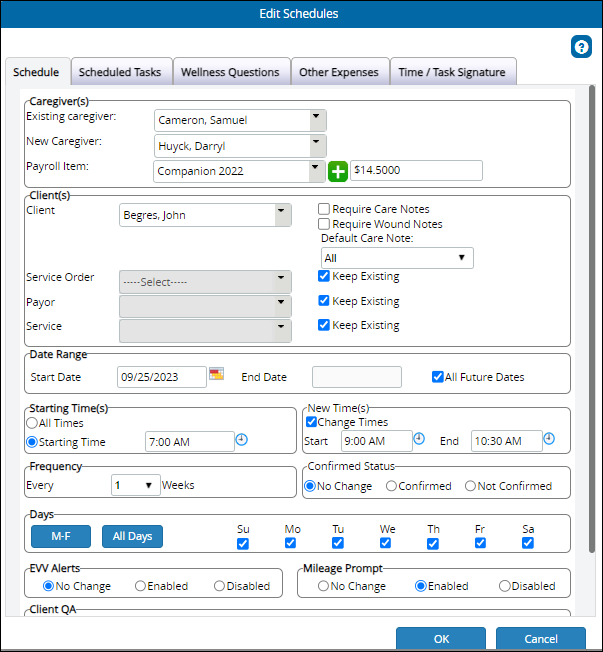Screenshot of a Scheduling App Interface:

The screenshot displays a scheduling application with the top section featuring a blue border. Within this blue border, the text "Edit Schedules" is prominently displayed in white. Below this header are several tab options including: "Schedule," "Schedule Task," "Wellness Questions," "Other Expenses," and "Time/Task Signature." The "Schedule" tab is currently selected.

In the "Schedule" tab, there are details about caregivers and scheduling specifics:
1. **Caregivers:**
   - **Existing Caregiver:** Cameron Samuel
   - **New Caregiver:** Hewick Darrell
   - **Payroll Item:** Companion 2022 plus $14,500

2. **Clients:**
   - **Client:** John Burgress
   - **Requirements:**
     - Require Care Notes: Unchecked
     - Require Wound Notes: Unchecked
     - Default Care Note: All

3. **Service Order:**
   - Payer: Service All Grade
   - Service Note: Keep Existing

4. **Date Range:**
   - **Start Date:** 09/25/2023
   - **End Date:** Blank (with "All Future Dates" checkmarked)

5. **Times:**
   - Starting Times: All Times
   - Specific Times:
     - 7 a.m. (Original Starting Time)
     - 9 a.m. (New Change)
     - 10:30 a.m. (New Change)

6. **Frequency:**
   - Every One Week

7. **Status:**
   - Confirmed Status: No Change
   - Options: Confirmed and Not Confirmed (with No Change selected)

8. **Days:**
   - Monday through Friday (Detailed Days: All Days Checkmarked)

9. **EW Alerts:**
   - No Change (Selected)

10. **Mileage Prompt:**
    - Enabled

Finally, at the bottom of the interface, there are two buttons: "OK" and "Cancel."